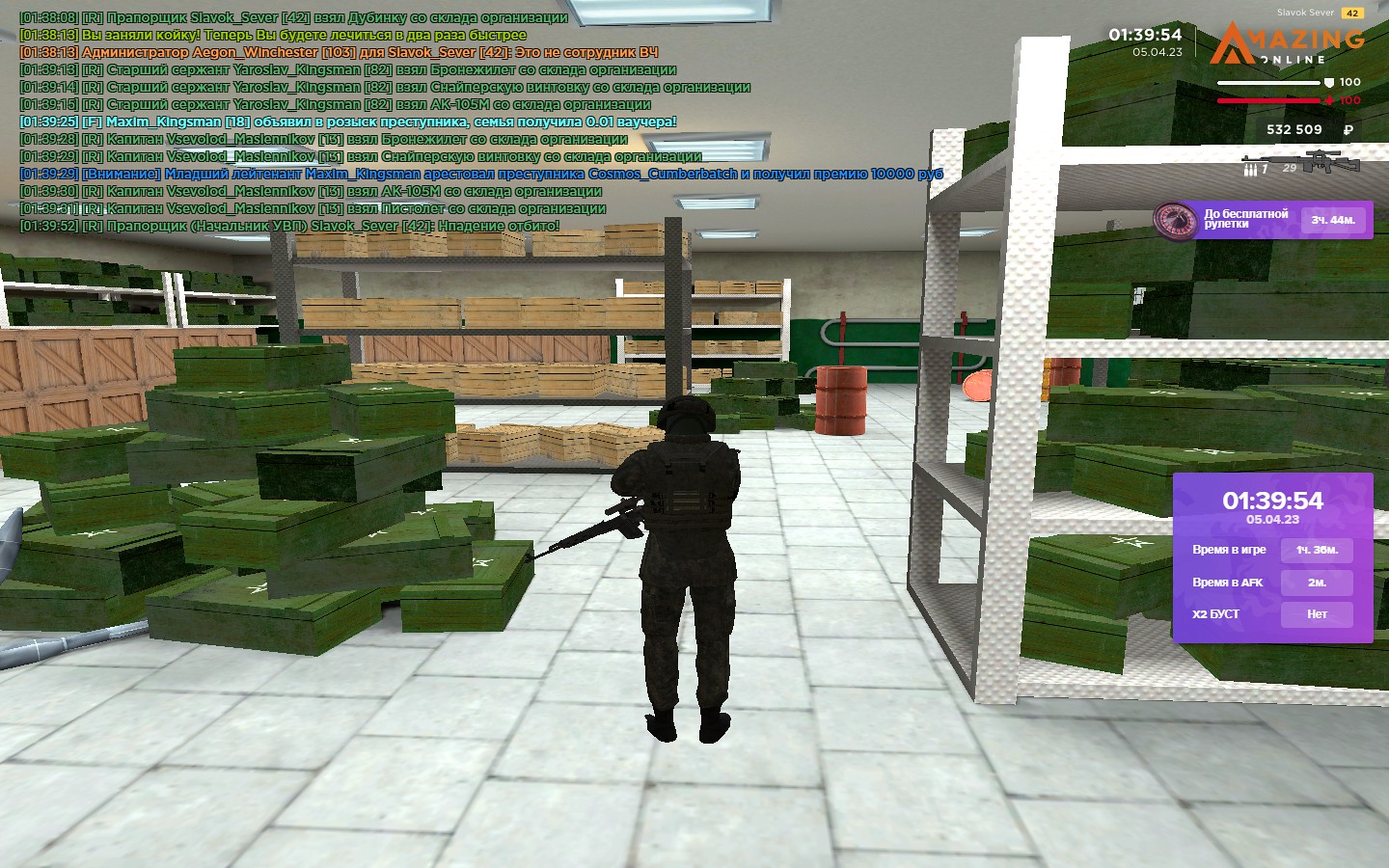The rectangular screenshot, oriented horizontally, appears to be from a first-person shooter video game. Dominating the foreground is a black silhouetted character, holding a rifle, and facing away from the camera. To the character's immediate left lies a stack of green boxes, complemented by additional green boxes on shelving to the right. The background features several racks of brown boxes, with some brown boxes seemingly beyond the frame. A notable red barrel stands amidst another pile of green boxes in the distance. The scene is set on a floor with gray tiling. 

In the upper left-hand corner of the image, small, hard-to-read text likely showcases player dialogue. On the right side, a time clock is present, displaying the text "amazing inline" along with the character's health stats, another score, and a weapon icon. Further information is provided in a smaller purple box, while a larger purple box features a time ellipse arc with indistinct numbers.